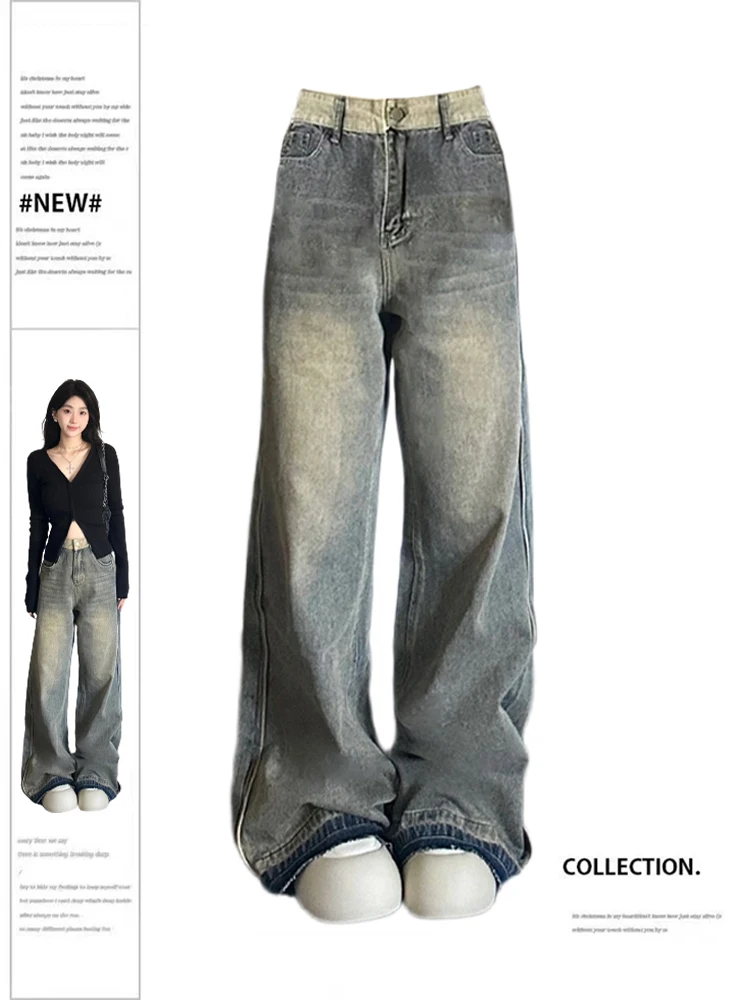The advertisement features a large photograph showcasing a pair of exceptionally baggy, pale grayish-blue jeans, with prominent fading down the thighs. At the top of the waist, the jeans have a white color, transitioning to gray around the pockets, and finishing with a dark blue tint at the ankle, resting over gray sneakers. A beige belt is threaded through the waist loops. Positioned on the bottom right of the image, the word "Collection" is displayed in black font. To the left, there's a rectangular inset featuring a full-view image of a young, Asian woman modeling the jeans. She has long, dark black hair, styled to fall behind her back. She dons a black, long-sleeved shirt that reveals her belly button and part of her chest, complemented by a silver cross necklace and a black strap across one shoulder, presumably from a purse or backpack. Above her are the words "New" in a bold caption, accompanied by several small black paragraphs, though the text is not legible.